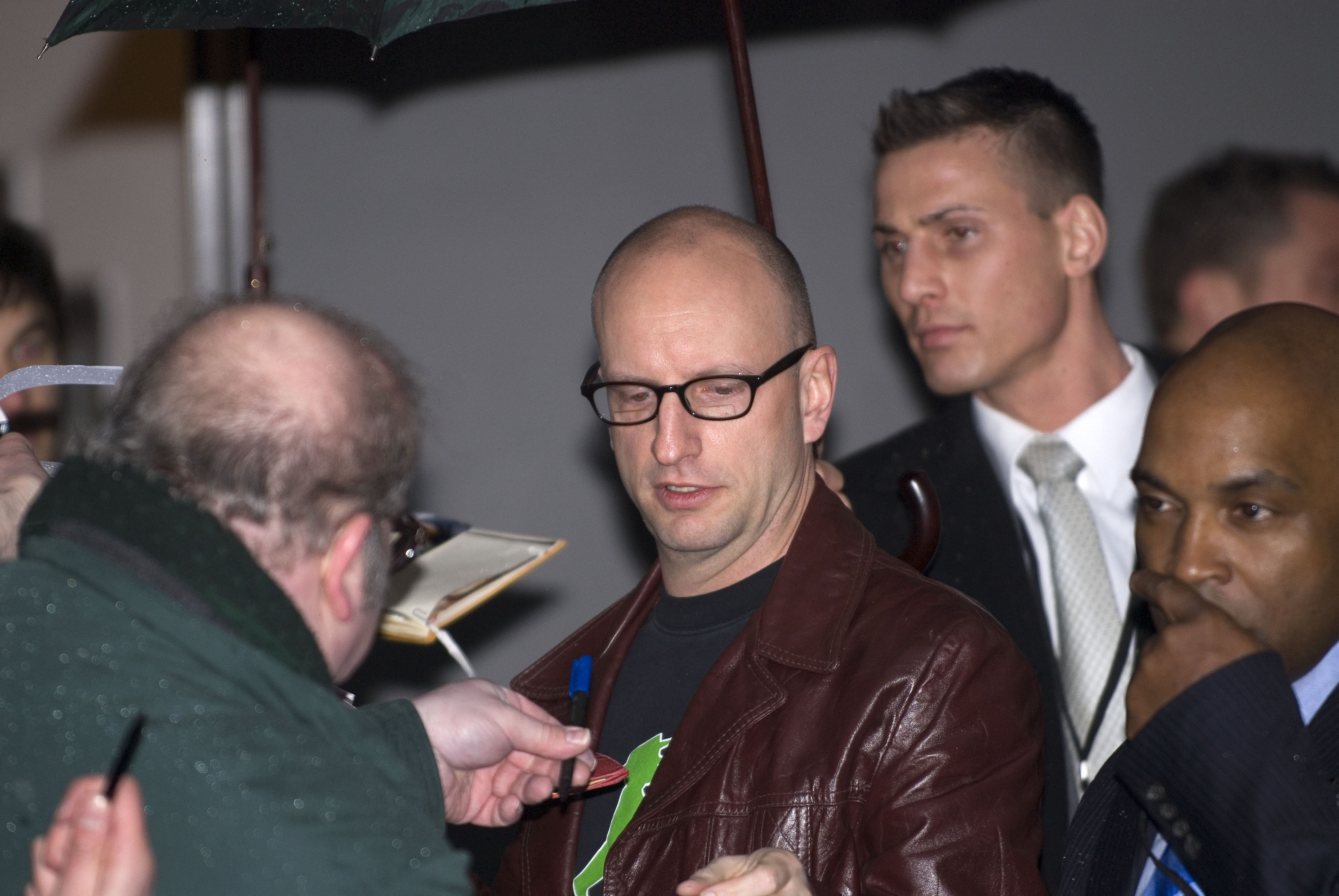In the photo taken at a press or signing event, a distinguished gentleman stands in the center, wearing black-framed glasses, a burgundy leather jacket, and a black t-shirt with a gray and green design. He appears to be someone of notable fame, engaging with individuals around him. To his left is an older man with light gray hair, dressed in a gray coat, holding a pen and seemingly requesting an autograph from the central figure. On the right side of the central man stand two bodyguards, one African-American and one white. The latter bodyguard, dressed in a dark suit, holds a black umbrella with a brown handle over the central figure. The background features a gray wall with silver elements, possibly poles, contributing to a somewhat industrial appearance. Additional people are partially visible; one in a blue pinstriped suit with a blue tie and white shirt, and another man wearing a brown leather coat and black undershirt with green details, also involved in the signing event.